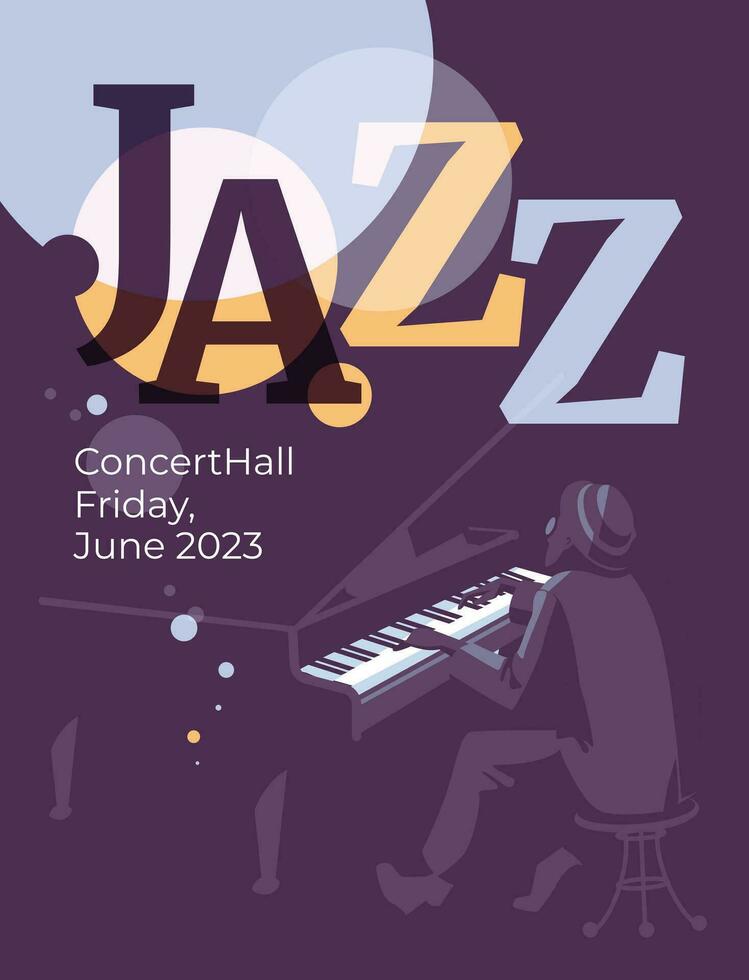The image is a promotional poster for an upcoming jazz concert in June 2023. The background is predominantly purple with decorative orange and blue elements. At the top, in large, colorful letters, the word "JAZZ" is prominently displayed, with the letters "JA" in purple, the first "Z" in orange, and the second "Z" in blue. Surrounding this text are various blue, white, and yellowish-orange bubbles and circles, adding to the vibrant aesthetic of the poster.

Below the word "JAZZ," there is a cartoon-style drawing of the silhouette of a man playing a piano. This silhouette is rendered in black and purple, making the figure easily distinguishable against the background. The piano in front of him features clearly visible white and black keys.

Further down the poster, additional text reads "Concert Hall, Friday, June 2023," positioned among smaller bubbles that echo the colors from the top of the poster. This detailed and colorful design unmistakably promotes a jazz concert, capturing attention with its lively and artistic presentation.